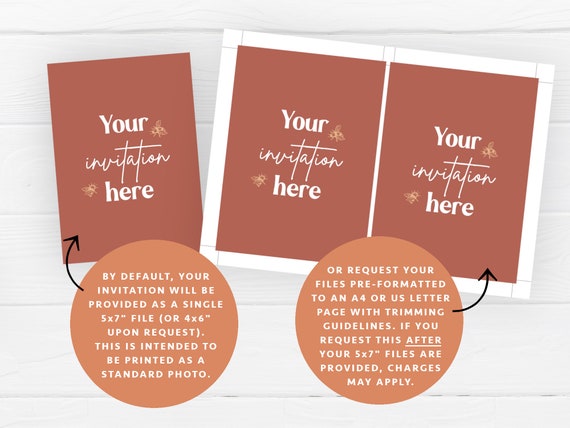This image is an advertisement for an online printing shop showcasing custom invitations. The setup is on a white, wood-grained background. The left side features a single, reddish-brown blank card with white text that reads "Your invitation here." This text is accompanied by small orange bees next to the letters "R" in "your" and "H" in "here." Below this card, a circle with an arrow pointing to the invitation states, "By default, your invitation will be provided as a single 5x7 file or 4x6 upon request. This is intended to be printed as a standard photo."

On the right, there is an image displaying a set of two similar brown invitations with white text, framed together with a white line separating them. An orange circle below these cards includes an arrow indicating, "Or request your files pre-formatted to an A4 or US letter page with trimming guidelines. If you request this after your 5x7 files are provided, charges may apply." This infographic highlights options for different formatting preferences and associated conditions.